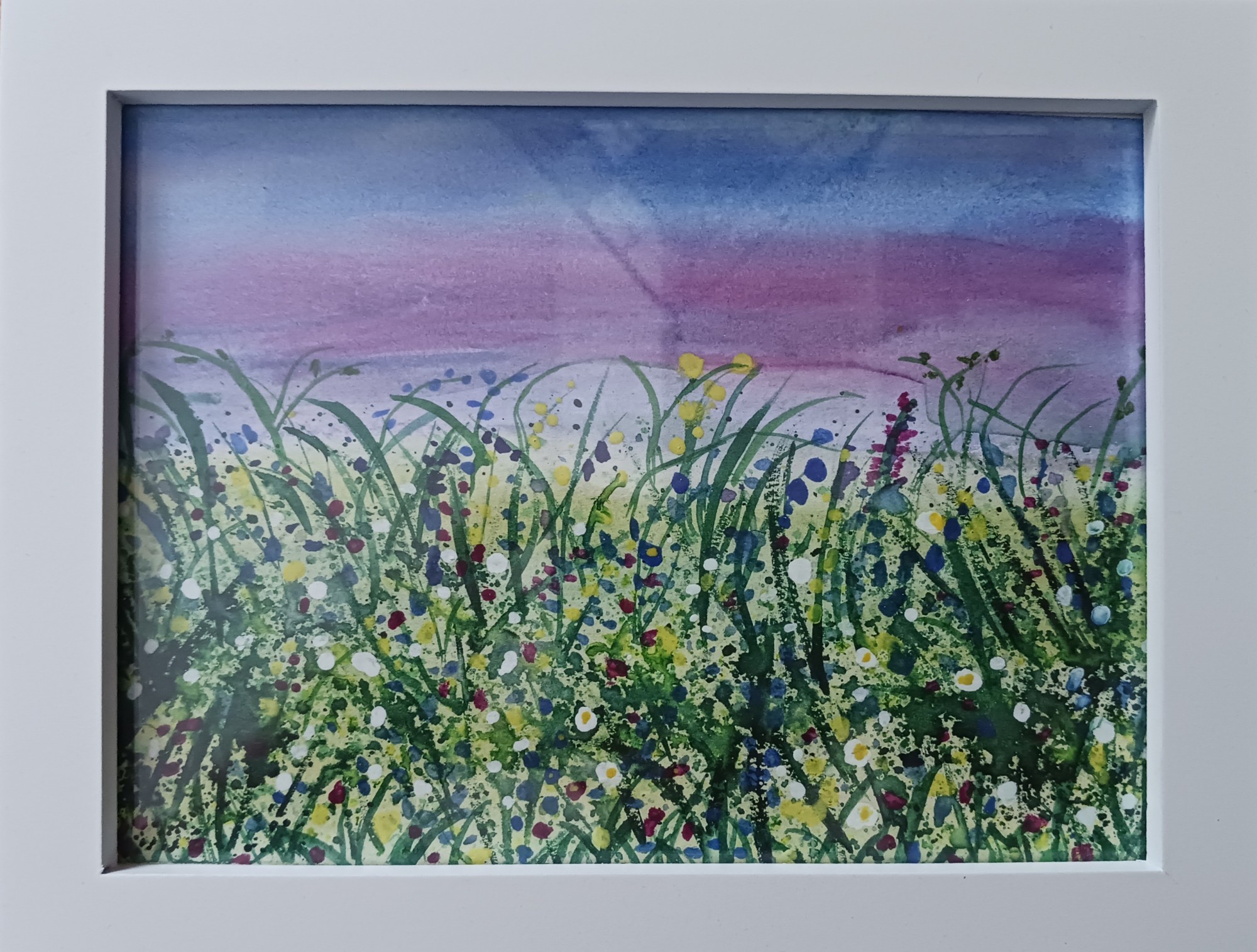The image depicts a lively, framed abstract painting of a vibrant field of wildflowers under a transitional sky. The bottom two-thirds of the painting are brimming with a dense assortment of vividly colored flowers and wispy grass fronds. Yellow, blue, indigo, magenta, red, white, and purple flowers, all small and numerous, create a mesmerizing tapestry of color. The flowers are rendered in a dot-like style, scattered haphazardly yet collectively forming the illusion of a thriving field. Long, green strands representing leaves interweave with the colorful petals, enhancing the impression of a living meadow. The background transitions from a blue sky at the top to a magenta-purple haze on the horizon, evoking the enchanting ambiance of a sunset or evening glow. This color-gradient sky occupies about forty percent of the painting, making the entire artwork feel alive and immersive.